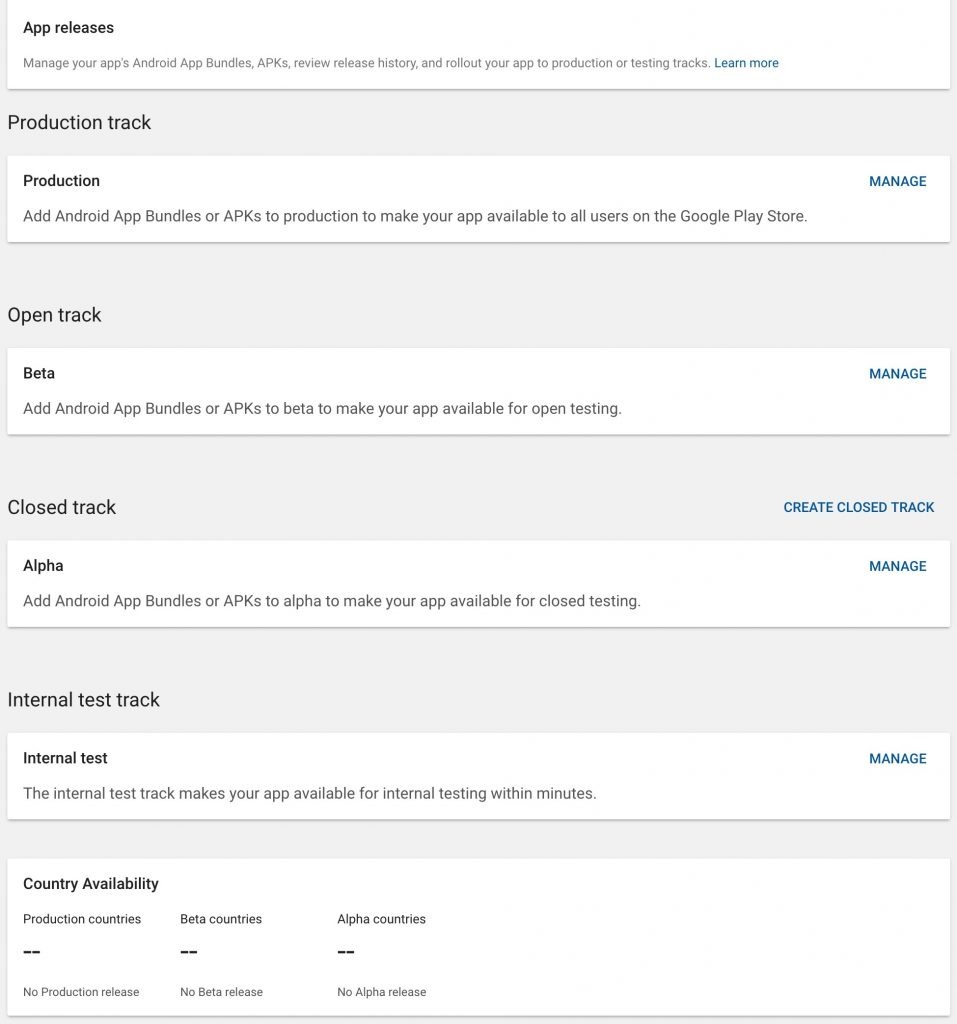A screenshot captures a website page dedicated to managing app releases and testing tracks on the Google Play Console. The interface showcases a predominantly white background accentuated with off-white borders that serve to distinguish various sections and options.

At the very top, a white panel titled "App Releases" provides multiple functionalities including managing apps, creating Android App Bundles, APKs, reviewing release history, and rolling out apps through production and testing tracks. A blue hyperlink labeled "Learn more" is prominently positioned here.

Directly below, the section labeled “Production Track” with an off-white border highlights the production phase of app release. The adjacent white panel on “Production” offers the option to add Android App Bundles or APKs to make the app available to all users on the Google Play Store. A blue "Manage" link is positioned to the right.

Continuing down, the "Open Track" is mentioned in another off-white border, leading to the "Beta" panel. This panel outlines adding Android App Bundles or APKs to the beta phase for open testing. A blue "Manage" link appears here as well. The off-white border also includes "Close Track" with the option "Create Closed Track" in blue.

Next, the "Alpha" panel within a white background specifies adding Android App Bundles or APKs for closed testing, accompanied again by a blue "Manage" link to the right. Below, another off-white border mentions "Internal Test Track," leading to the "Internal Test" panel which describes making the app available for internal testing within minutes, and another blue "Manage" link is to the right.

Finally, at the bottom of the page, the "Country Availability" section lists "Production Countries," "Beta Countries," and "Alpha Countries," all marked with double negative check marks indicating that no releases have been made in any of these categories. Detailed mentions include "No production released" under Production, "No beta release" under Beta, and "No alpha release" under Alpha respectively.